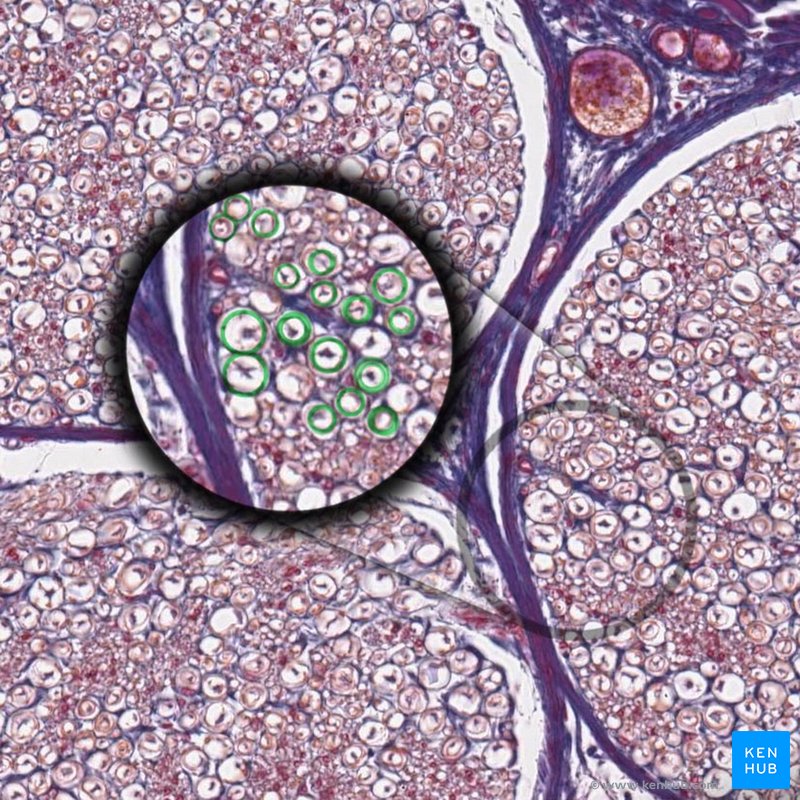This highly detailed microscopic image, sourced from Kenhub, showcases a histological sample that likely presents blood cells or a similar cellular structure. Dominated by pinkish-purple hues, the image features three primary large lobes filled with numerous smaller cells. Within these lobes, a magnified portion is highlighted, outlined in black to accentuate the cellular details. This magnified area reveals a smaller circle attached to it, reminiscent of a reel-to-reel player, and calls attention to specific cells using green circles, possibly indicating unique or noteworthy characteristics, such as deformation or disease. Additionally, in the top right and bottom right corners of the image, there are smaller lobes and a detailed smaller highlighted circle, which further elaborates on the cellular composition. The name "Kenhub" appears in the lower right corner, providing the source of the image.